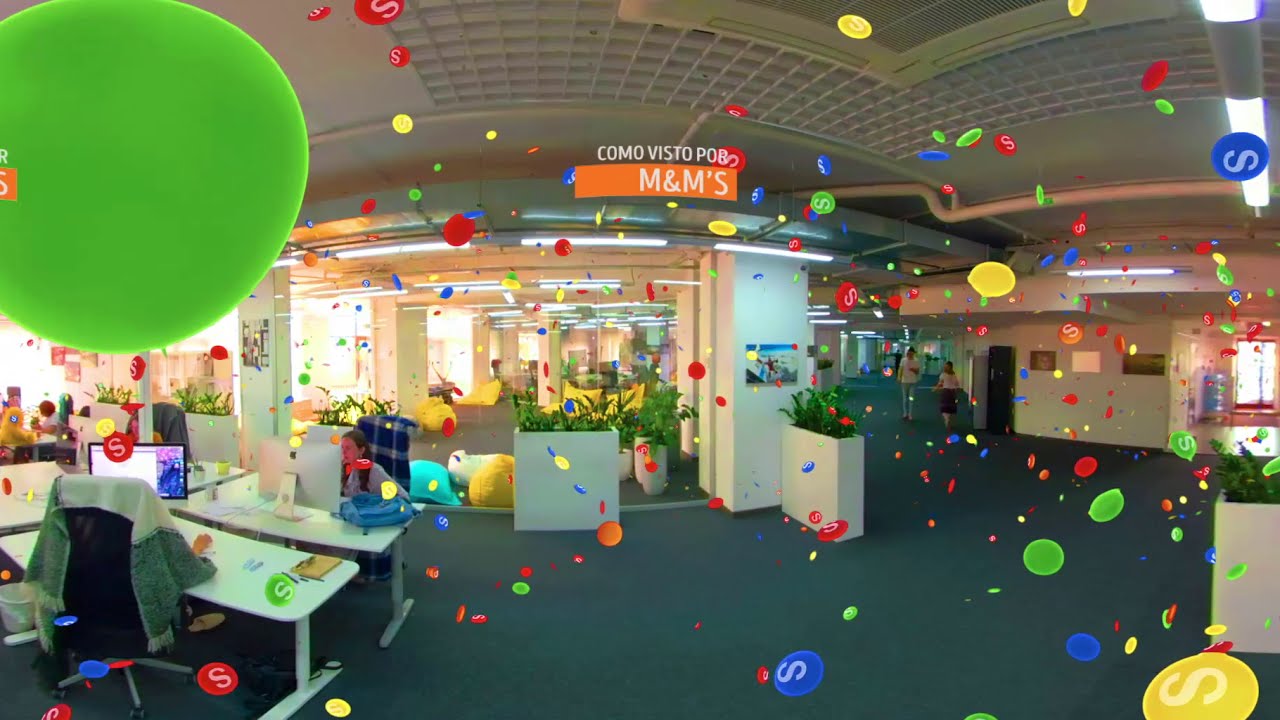This intriguing and vibrant image appears to be a digitally enhanced photograph or AI-generated composite of a modern office lobby or vestibule, potentially in a Spanish-speaking region. At its center, a red strip featuring the words "Como Visto" and "P.O.B." next to "M&M's" suggests it might be an advertisement. The setting is bright and colorful, with a modern aesthetic characterized by white walls, white pillars, and navy blue flooring. The scene includes various office features like white desks, beanbag chairs, plants, and several people including a woman seated and others walking through the space. A water jug and illuminated signage also add to the office environment.

What stands out is the overlay of vibrant, confetti-like objects resembling M&Ms or Skittles, in green, yellow, blue, and red colors, intriguingly marked with the letter "S" instead of the traditional "M." These cylindrical shapes are scattered throughout the image, creating a festive, surreal atmosphere. The overall impression suggests a playful, high-spirited advertisement within a dynamic office lobby setting.